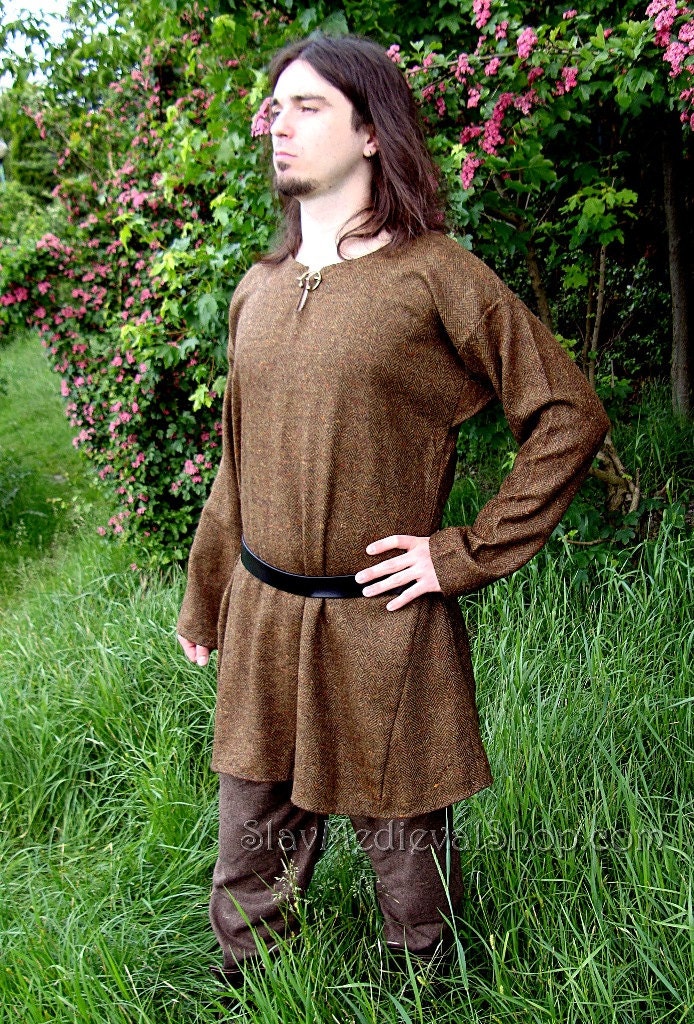In the photograph, a young man stands in a knee-high grassy field near a small forest. He wears a brown, medieval-style tunic that extends halfway down his thighs, secured with a black leather belt. His attire includes simple, dark woolen pants. His left hand rests on his hip while his right arm hangs by his side. He has shoulder-length dark hair and a slightly rugged appearance with a goatee and soul patch. His complexion is very pale, and he sports an ear piercing. Notable is a decorative metal pin at the neckline of his tunic, possibly used to keep it closed. Behind him, a bush adorned with purple and pink flowers adds a touch of color to the scene. The image has a watermark indicating "slavmedievalshop.com," suggesting the attire is from a themed shop.